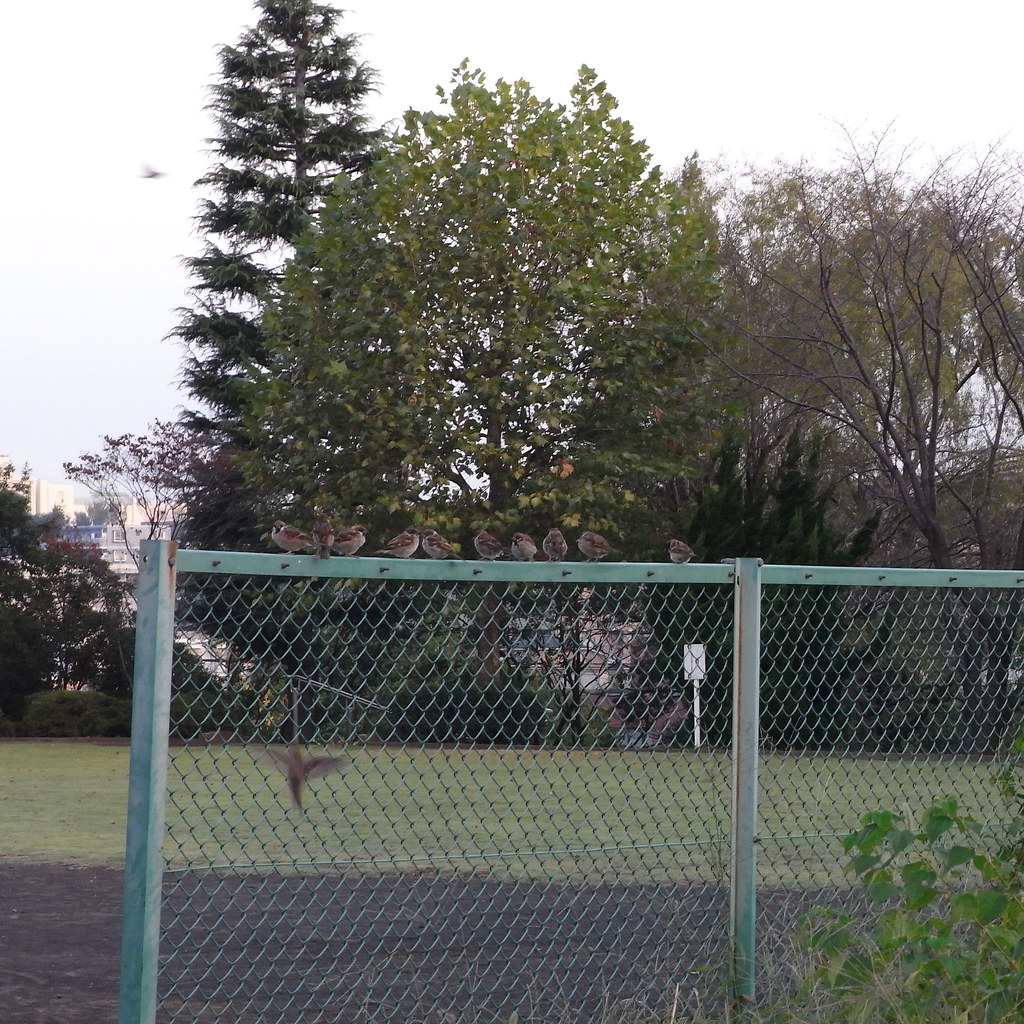In the foreground of the image, a green chain-link fence with green poles stretches across, with an opening on the left side. Perched on the top horizontal rail of the fence, there are about ten small, brown birds, some with hints of gray on their stomachs, all facing the camera. One bird is captured in flight, blurry due to motion, as it descends toward the fence. 

Behind the fence, a mix of greenery and bare spots create a varied backdrop. There is a strip of green grass, transitioning into patches of dirt. To the right of the fence, some weeds are visible, while the lower right corner features a small, green bush.

Further back, a variety of trees populate the scene. A tall, skinny, green tree stands beside a round, leafy tree, and a third tree with sparse leaves and visible branches helps create depth. The background also reveals trees that are fully green and others that are bare. 

In the distance, on the left, a small bird is seen flying. Beyond the trees, to the left side, the vague outlines of buildings can be discerned. The sky, mostly obscured and appearing almost white with slight touches of blue, frames the upper portion of the image. A white sign with a white post can be spotted amidst the vegetation. The overall scene is serene, capturing a quiet moment in this natural, yet slightly urban environment.